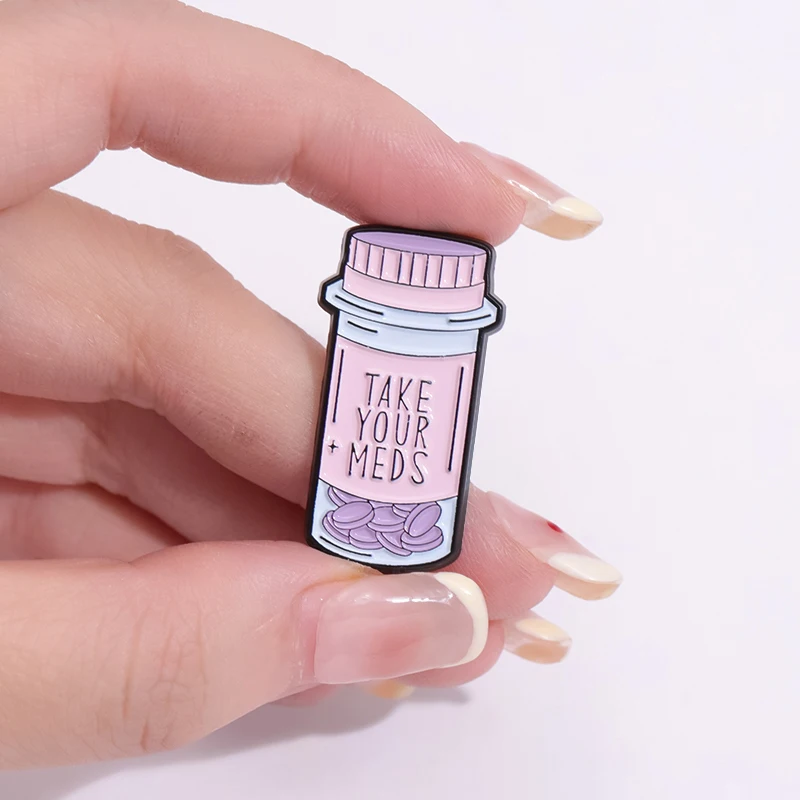The image showcases a close-up of a pale white woman's hand with a French manicure, although her nail tips have noticeably grown out and need a refill. The hand, positioned against a white background, is holding a small acrylic pin with her index finger and thumb. This pin is shaped like a pill bottle, featuring a blue body with a pink label in the middle and a pink and purple cap. The label reads "Take your meds" in black lettering. Purple, round pills with black outlines can be seen at the bottom of the bottle design. The pin's details and the shadow cast by the hand suggest it could be an advertisement, potentially for a handmade marketplace like Etsy.